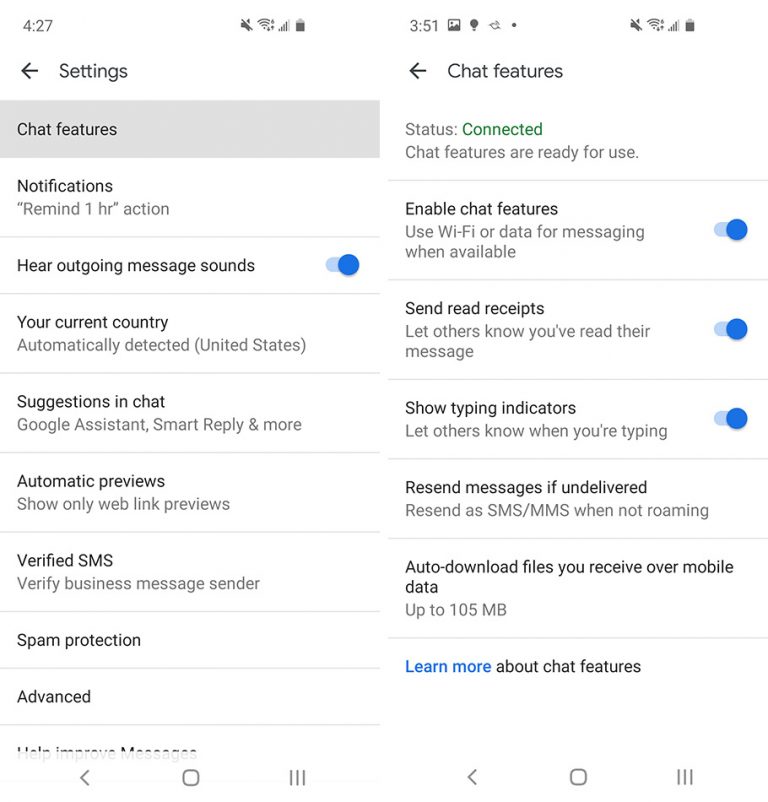The image showcases two mobile screenshots displayed side by side with different timestamps—4:27 on the left and 3:51 on the right, indicated at the upper left-hand corner of each screenshot. Both screenshots feature chat settings. The top left corner of the left-hand screenshot reads "Settings," while the top left corner of the right-hand screenshot reads "Chat Features."

Each screenshot consists of a list within horizontally arranged white background sections, highlighting various toggles for chat features. Both images display four blue-enabled slider bars, indicating that specific features are turned on. The activated features on both screens include:
- Hear outgoing message sounds
- Enable chat features
- Use Wi-Fi data for messaging when available
- Send read receipts, letting others know you've read their message
- Show typing indicators, letting others know when you're typing

Both screenshots also feature a set of icons at the top and bottom sections. Additionally, a green label indicating "connected status" and a blue "learn more" link are visible at the bottom left-hand corner of the right screenshot.